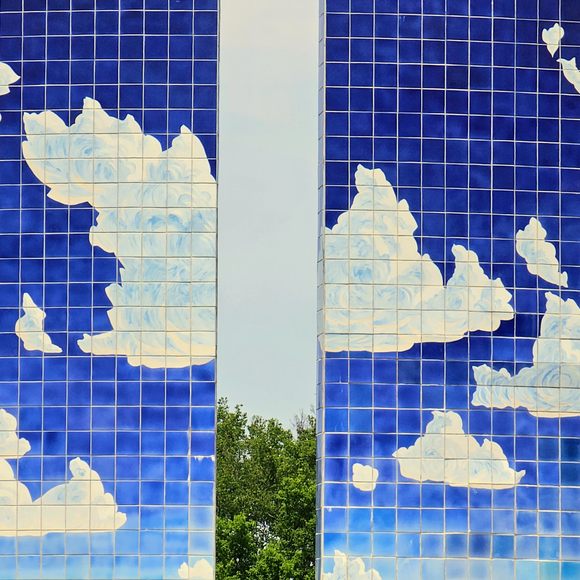The image captures a detailed and decorative monument consisting of two large, rectangular obelisks that stretch from the bottom corners to the top corners of the frame, with a narrow gap between them. This gap reveals a light gray sky above and tree branches adorned with green leaves at the bottom. Both obelisks, partially out of frame, are intricately covered with blue painted porcelain tiles featuring white fluffy clouds at random intervals, mimicking the open sky. The obelisks give the image a mosaic-like appearance with varying shades of dark and light blue interwoven with the clouds, suggesting a blend of artistic representation and natural elements. The central vertical sliver in the image showcases a photographic strip of the actual sky and tree tops, contrasting the painted mosaic tiles on either side. The tiles, joined by white grout, collectively create a surreal blend of painted and real sky imagery, enhancing the monument's artistic and serene appeal.